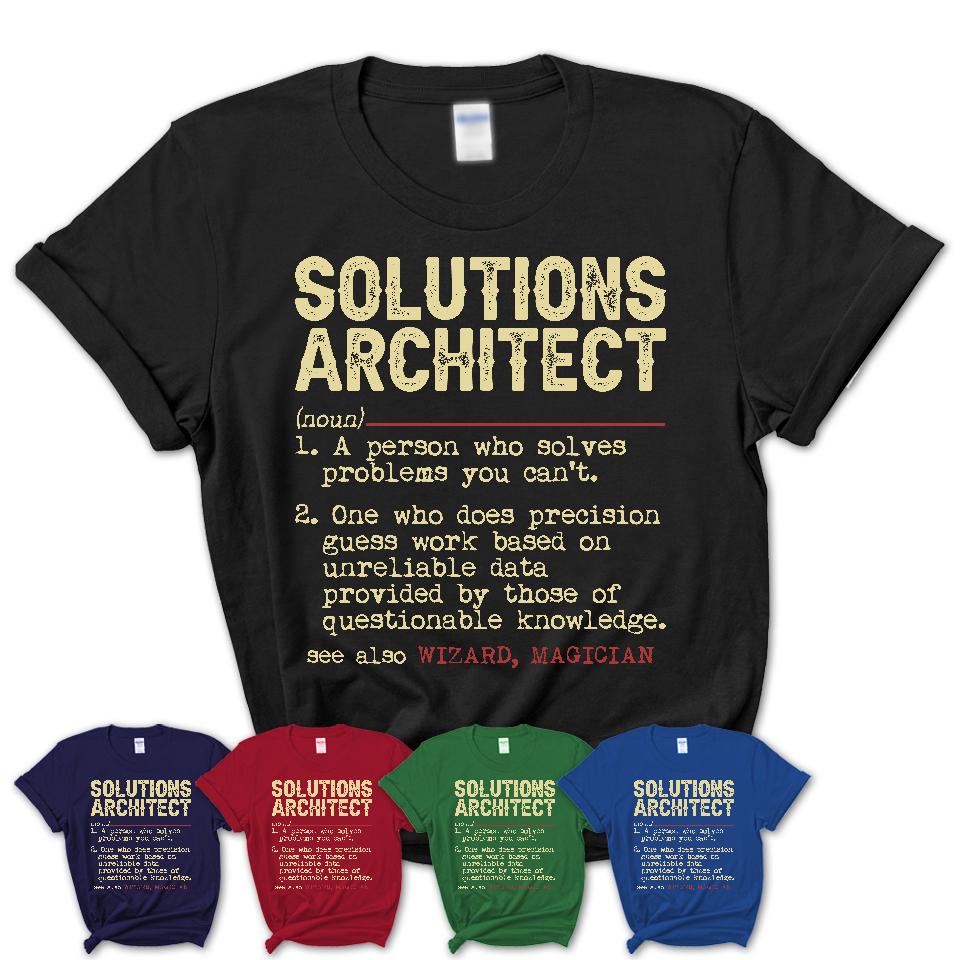The image features a series of t-shirts displayed against a white background, with the primary focus on a black t-shirt and several smaller variations underneath. The t-shirts come in five colors: black, navy blue (almost purple), red, green, and a lighter blue. Each t-shirt is adorned with text in a dictionary-style format. In bold, the text reads "Solutions Architect" followed by "noun" in lighter yellow font. The definition includes two points: "1. A person who solves problems you can't. 2. One who does precision guesswork based on unreliable data provided by those of questionable knowledge." In red, smaller text adds, "See also: wizard, magician." The black t-shirt stands out prominently, while the smaller color variations are neatly arranged below it, highlighting the diverse color options available for this design. Additionally, a white care tag can be seen at the neckline of each t-shirt.